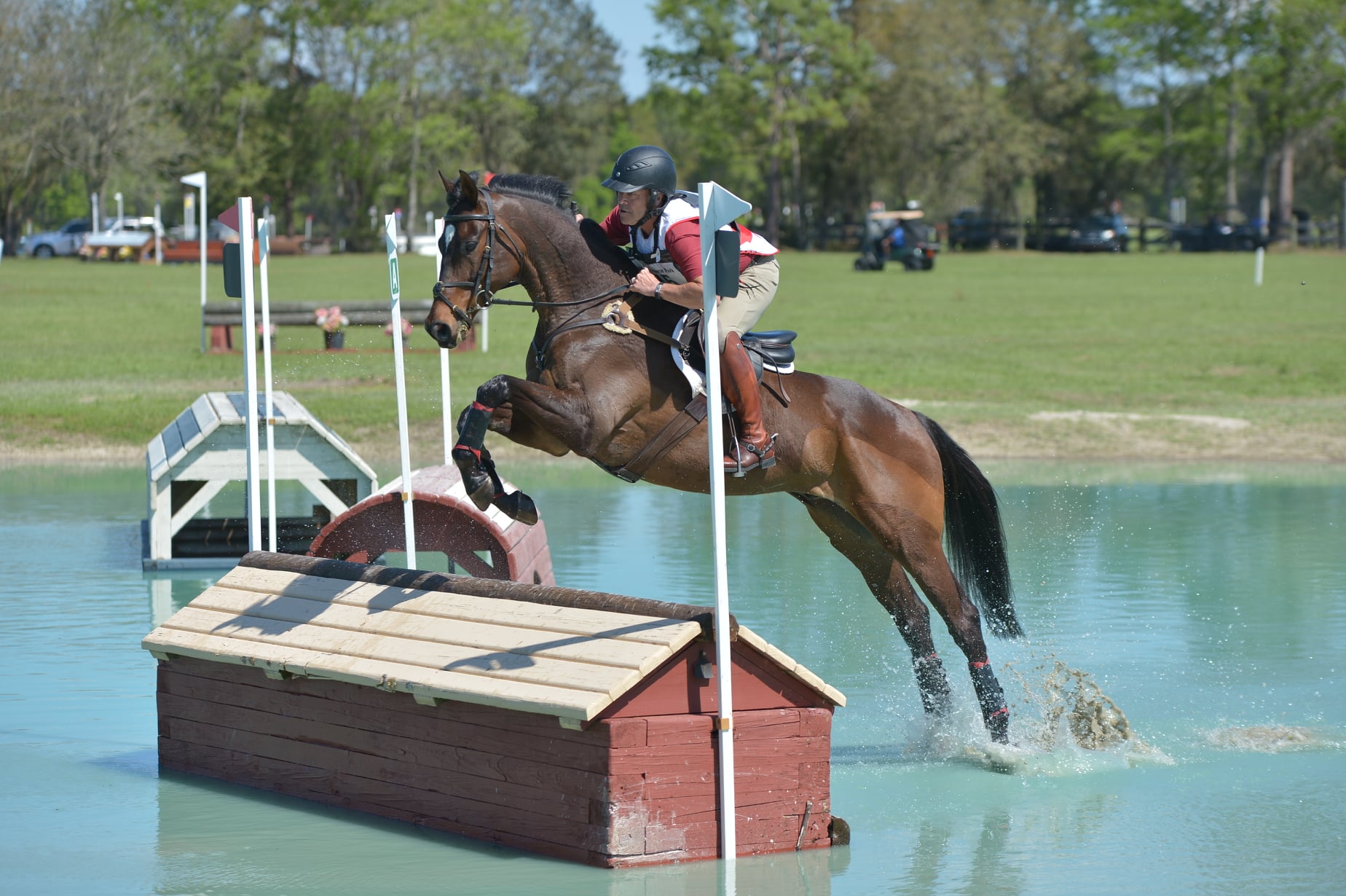This vibrant, professional photograph captures a dynamic moment at an outdoor equestrian event on a bright, sunny day. The image, possibly a video freeze-frame, is set in a picturesque landscape orientation. The background is framed by lush green grass and a dense cluster of dark green trees under a clear blue sky, indicating a season other than fall. A few out-of-focus vehicles in colors such as yellow, white, and blue are parked just beyond the edge of the grassy field.

The foreground features a shallow water obstacle, around a few inches deep, with a distinctive low structure resembling a red barn with a cream-colored roof. This obstacle is flanked by two white poles, creating a challenging barrier for the competitors. The central focus is a striking dark brown horse with a flowing black mane and tail, captured mid-jump as it deftly clears the obstacle. The horse’s front legs are raised and its powerful rear legs are still splashing in the water below. 

Riding the horse is a female jockey, perfectly poised in a jump position. Additional water obstacles are visible in the background, enhancing the complexity of the equestrian course. This photo exemplifies photographic realism, freezing a moment of athletic grace and synchronization between horse and rider in a scenic, natural setting.